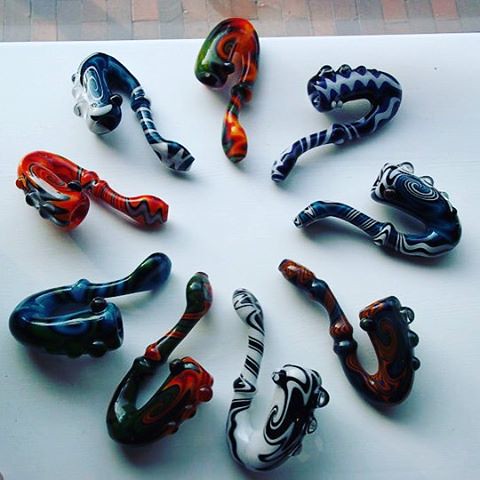This square color photograph features a collection of nine decorative, hand-blown glass pipes arranged artistically in a circle on a white surface, likely a table. Beyond the table, there's a thin strip at the top of the frame showing light pinkish bricks, possibly indicating a sidewalk or paving outside a shop window. Each pipe is uniquely designed and colorful, resembling mini saxophones, with their stems pointing inward. The pipes, adorned with decorative glass knobs and swirls, display a variety of colors: 

- A red and black pipe.
- A black and white one.
- A pipe with red and blue stripes.
- Another with a blue and black pattern.
- A red pipe with blue decorative blobs.
- A black or dark blue one with clear glass bumps.
- A blue and white striped pipe.
- A red pipe with bumps along its side.
- A dark brownish-red one with bumps.

Overall, the photograph captures the modern, intricate artistry of these smoking pipes against a clean, white backdrop, without any text to distract from their visual splendor.